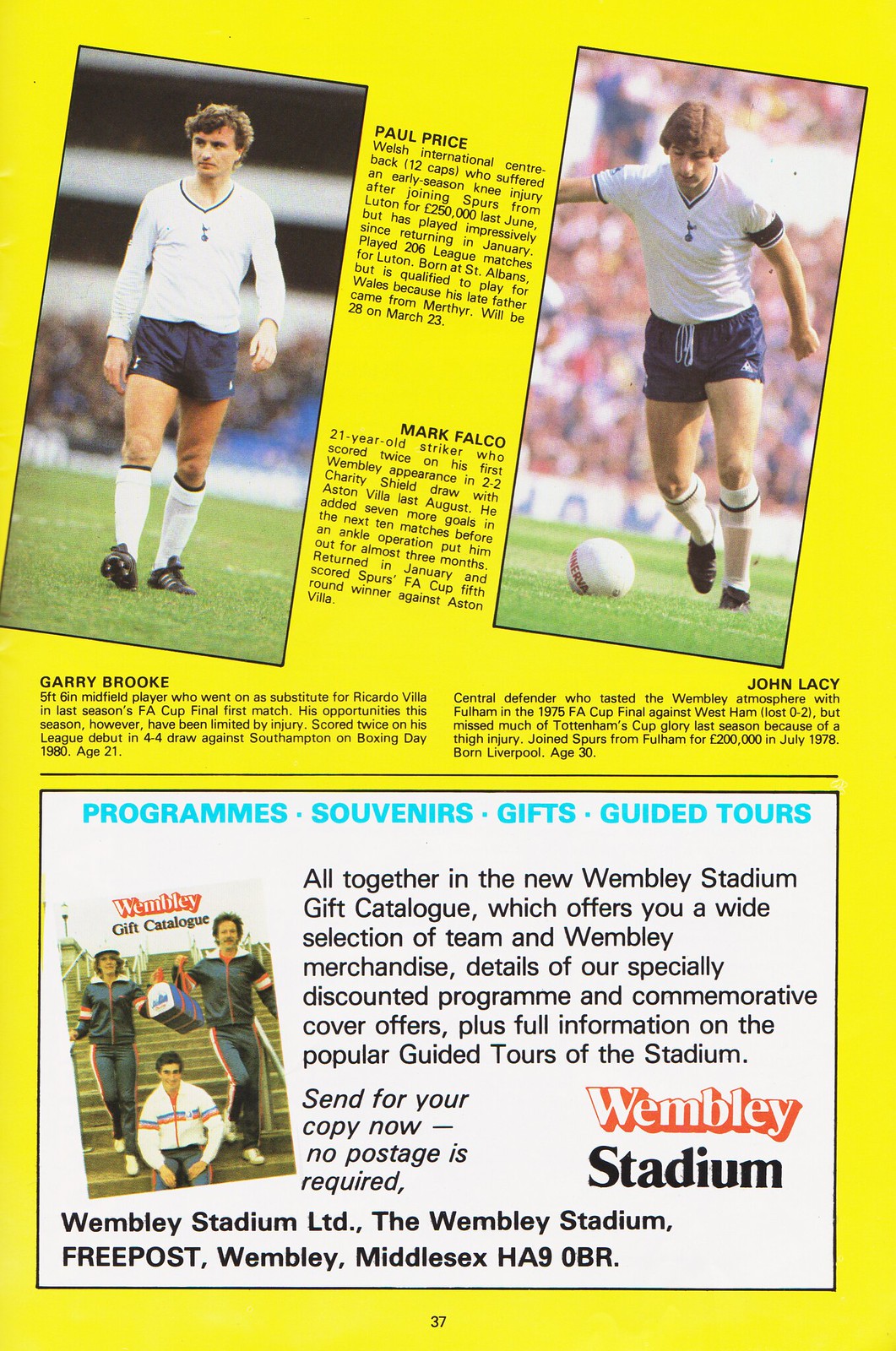This vertically aligned rectangular image appears to be a page from a soccer magazine, set against a solid yellow background and marked as page 37 at the bottom. At the top, there are two slightly slanted vertical rectangular pictures of soccer players, set against the blurred backdrop of stadium stands. The left image features Paul Price, identifiable by his brown hair, navy blue shorts, white tall socks, white long-sleeve shirt with a blue-striped collar, and black cleats as he walks across the grassy field. The right image shows Mark Falco in the same uniform, short-sleeved, running with a white soccer ball poised for a kick. Between these pictures, there's descriptive text about both players. Below this, Gary Brooke and John Lacy are also mentioned with brief descriptions, though their images are not shown. The lower part of the page includes a large rectangle with a white background and black border displaying promotional information. It advertises programs, souvenirs, gifts, and guided tours from the new Wembley Stadium Gift Catalog, which showcases an image of a magazine cover featuring three players standing on stairs, and provides details about merchandise and special offers. The entirety of the image is filled with these elements, making it a detailed and vibrant representation of a magazine page dedicated to soccer and Wembley Stadium memorabilia.